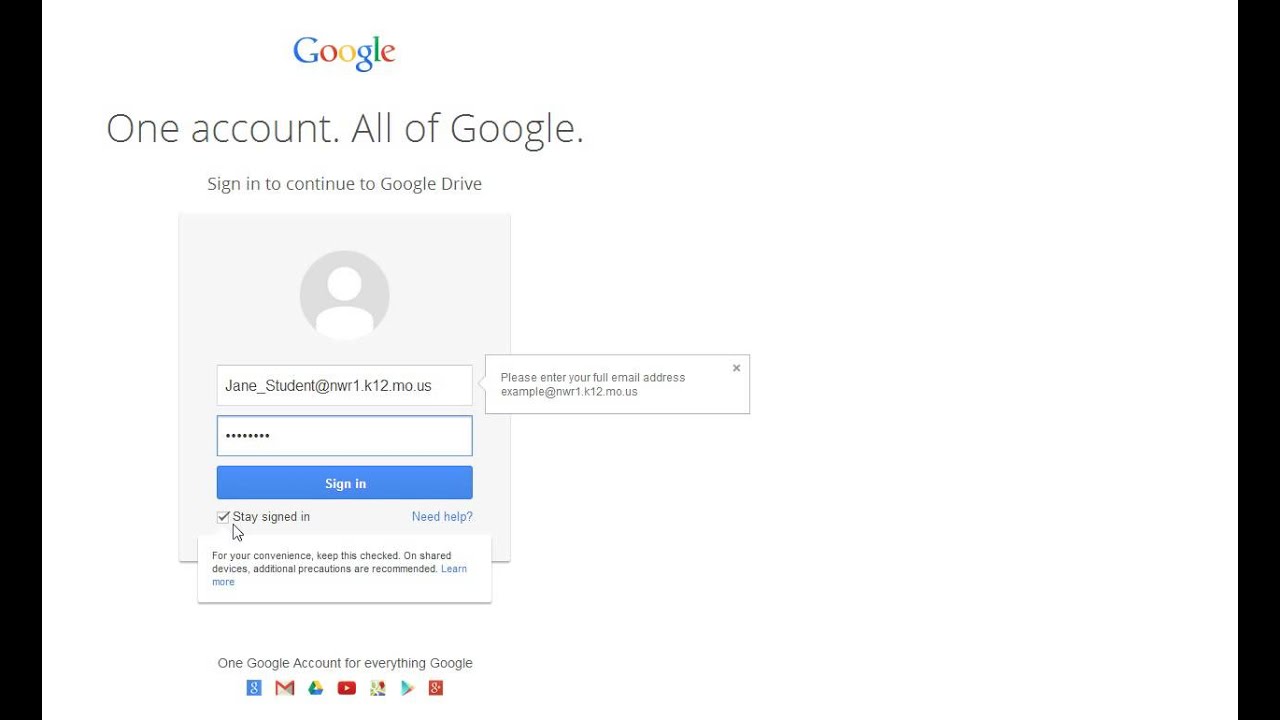This screenshot captures the Google login page, characterized by its crisp and clean design. At the very top is the iconic, multi-colored Google logo. Directly beneath it, a prominent title reads, "One account. All of Google." in large, bold text. This sets the stage for users to either log in or create an account. Beneath the title, the prompt "Sign in to continue to Google Drive" indicates the specific Google service to access.

Central to the screen is the user profile icon, currently displaying the default empty icon, signaling no active user. Following this, input fields await the user's login credentials, specifically requesting an email address and password. 

Just below these fields, the blue "Sign In" button stands out, ready to facilitate user entry once credentials are provided. Adjacent to it, a checkbox offers the option to "Stay signed in" for user convenience, with a tooltip explanation appearing when hovered over. This pop-up reads, "For your convenience, keep this checked. On shared devices, additional precautions are recommended.", accompanied by a "Learn more" link for further information.

To the right of the "Stay signed in" option, a "Need help?" link is readily available for users requiring assistance. At the bottom of the page, a series of Google icons form a visual reminder of the extensive reach of a single Google account, underlining the text, "One Google account for everything Google."